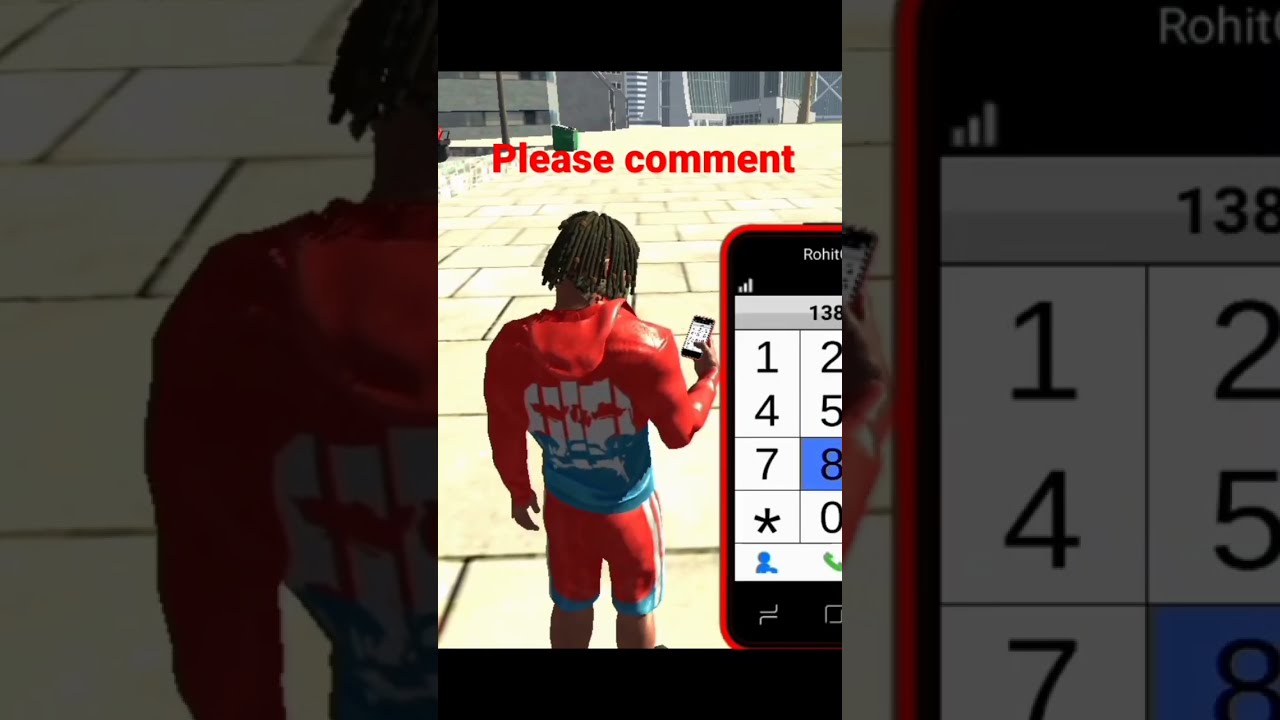The image prominently features a central figure that appears to be a teenage boy, possibly a character from a video game. He is dressed in a noticeable orange football uniform with white stripes and additional padding that makes him look more muscular. The uniform includes a long-sleeved jacket with intricate designs on the back, resembling either a skull or a decorative pattern, and red and white shorts. The character has shoulder-length dreadlocks and is looking down at an iPhone, notably pressing the number 8. The setting appears to be a sunlit city street, with a beige concrete pavement and distant skyscrapers. Surrounding the central image are fragmented, enlarged, and slightly faded excerpts of the same picture on the left and a close-up of the iPhone screen on the right. The entire composition mimics the shape of a high-definition television screen. At the top of the image, the text "please comment" is displayed in red, further indicating an interactive or digital context like a video game interface or social media post.